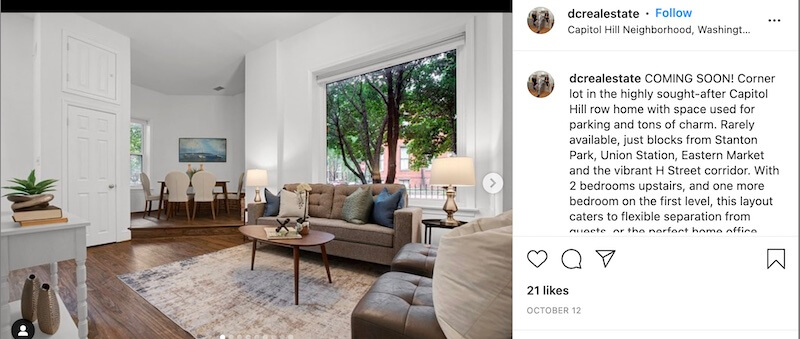This is a screenshot from a social media platform, possibly Instagram. The image is landscape-oriented and is set against a white background with a thin black line bordering the right side. 

On the left side of the screenshot, there's a photo of a stylish living room with dark brown hardwood flooring. The room features an elevated area with a brown table and white chairs, accompanied by a painting in the background. Centrally positioned is a long table, surrounded by a sofa and leather chairs. To the right of the sofa, there is a side table with a lamp. The room is illuminated by natural light streaming through a large window, offering a view of a tree outside.

To the right of the living room photo, there’s a text section laid out in a portrait orientation against a white background. The text includes an avatar (not clearly discernible) of a user named "DC Real Estate," followed by the option to follow them. The post's heading reads "Capitol Hill Neighborhood, Washington."

Below this, a thin border separates the introductory text from the detailed comments, which read: "Coming soon, corner lot in the highly sought after Capitol Hill row home with space to use for parking and tons of charm. Rarely available, just blocks from Stanton Park, Union Station, Eastern Market, and vibrant 8th Street Corridor. With two bedrooms upstairs and one more bedroom on the first level, this layout caters to flexible separation." 

The post is interactive, displaying options to like, share, and comment on the content. It has garnered 21 likes.